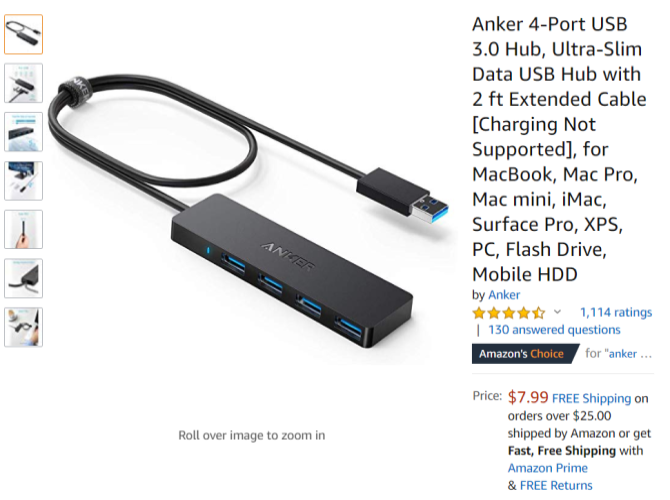This image is a detailed screenshot from the Amazon website, capturing a product listing for an Anker 4-Port USB 3.0 Hub. The screenshot is in a square format, resembling a picture taken from a laptop or computer screen. The central area of the image displays a gray rectangular USB hub with light blue port interiors, accompanied by a looping wire ending in a USB connector with a gray or silver tip and blue interior.

To the left of the product image, there is a comprehensive description which reads: "Anker 4-Port USB 3.0 Hub, Ultra-Slim Data USB Hub with 2-Foot Extended Cable, Charging Not Supported for MacBook, MacBook Pro, MacBook Mini, iMac, Surface Pro, XPS, PC, Flash Drive, Mobile HDD by Anker." Below this, it shows a user rating of approximately 4.5 out of 5 stars from 1,114 ratings, along with 130 answered questions. The "Amazon's Choice" badge is also prominently displayed below the star rating, within a dark blue box where "Amazon" is in white and "Choice" is in orange.

Further down, the price is marked as $7.99 in a prominent reddish-orange font, and there's a note about free shipping on orders over $25. Along the left margin of the main product photo, there is a vertical column comprised of seven thumbnail images, allowing viewers to preview additional product photos by hovering over them.